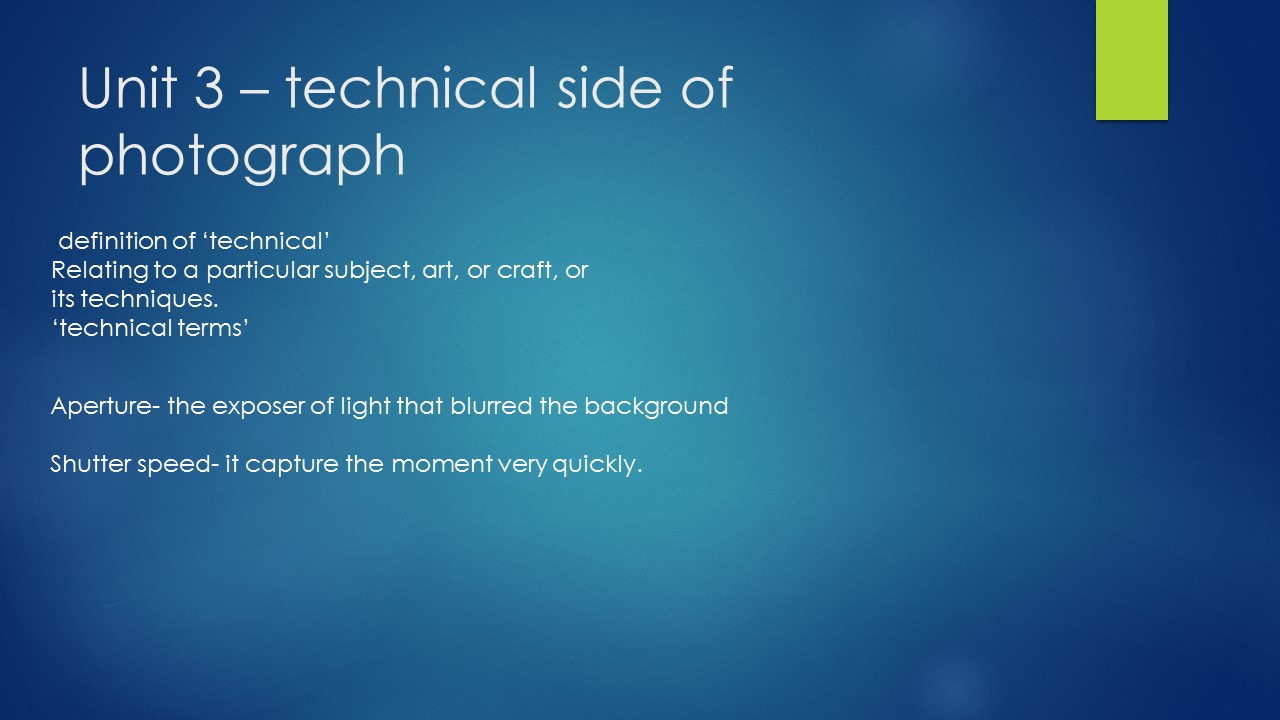The image is of a PowerPoint slide designed for an educational presentation on photography, specifically titled "Unit 3 - Technical Side of Photograph." The slide features white text concentrated toward the top left quarter of a blue background, which transitions to a brighter blue in the center, possibly mimicking sunlight. In the top right corner, there's a tall, narrow, yellowish rectangle adding a design element to the slide. The main heading, "Unit 3 - Technical Side of Photograph," is prominently displayed in large text. Beneath it, in smaller text, several points are listed: 

- "Definition of Technical (relating to a particular subject, art, or craft, or its techniques)"
- "Technical terms,"
- "Aperture - the exposure of light that blurred the background"
- "Shutter Speed - it captures the moment very quickly."

This slide serves as an introductory overview of the technical aspects of photography, covering key concepts such as aperture and shutter speed.